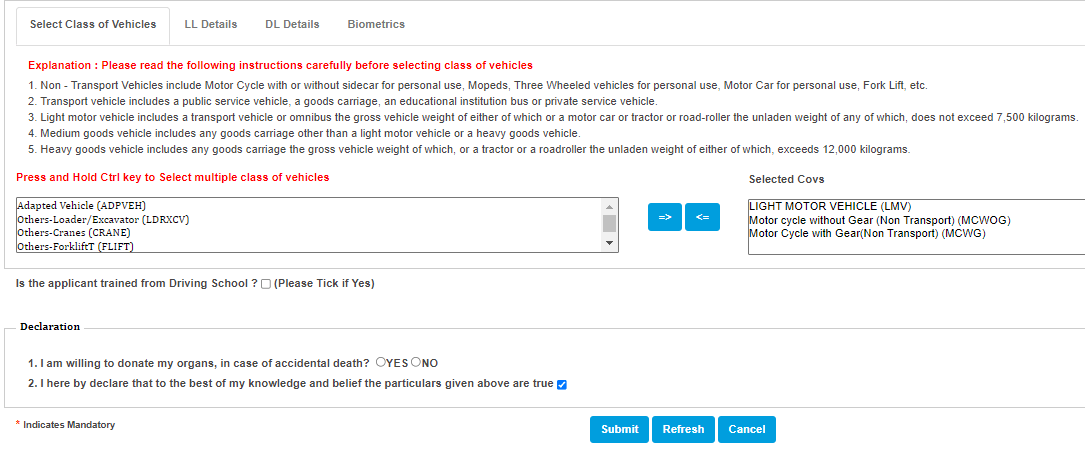The image is a screenshot of a website focused on vehicle information and categorization. At the top of the webpage, there are four tabs aligned horizontally: "Select Class of Vehicles" (which is the currently active tab), "LL Details," "DL Details," and "Biometrics."

Under the "Select Class of Vehicles" tab, a prominent red-font header reads, "Explanation: Please read the following instructions carefully before selecting class of vehicles." Beneath this header, the documentation is presented in standard black font, enumerated from 1 to 5:

1. **Non-Transport Vehicles:** Includes motorcycles with or without sidecar (for personal use), mopeds, three-wheeled vehicles for personal use, motor cars for personal use, forklifts, etc.
2. **Transport Vehicles:** Encompasses public service vehicles, goods carriages, educational institution buses, and private service vehicles.
3. **Light Motor Vehicles:** Comprises transport vehicles or omnibuses with a gross vehicle weight not exceeding 7,500 kilograms, as well as motor cars, tractors, or road rollers with unladen weights not exceeding the same limit.
4. **Medium Goods Vehicles:** Covers any goods carriage other than light or heavy goods vehicles.
5. **Heavy Goods Vehicles:** Includes goods carriages with a gross vehicle weight exceeding 12,000 kilograms, as well as tractors or road rollers with unladen weights over that threshold.

Below these instructions, there are several actionable buttons labeled "Is Applicant Trained from Driving School," along with options for submitting, refreshing, and canceling the information input.